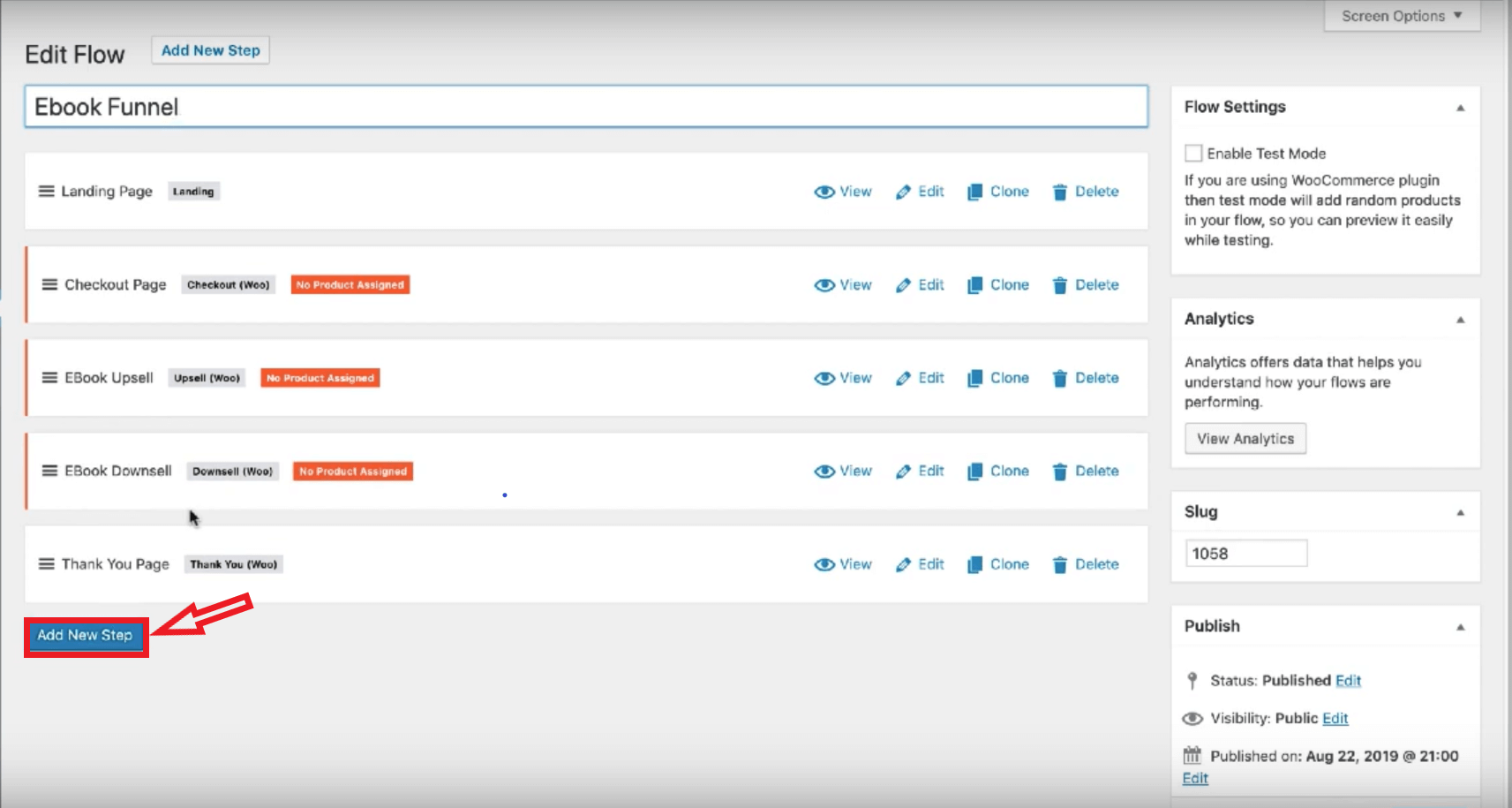Screenshot Description: 

The screenshot features a gradient background transitioning from gray at the top to light gray at the bottom. Positioned in the top left corner, the text "Edit Flow" is displayed prominently. Adjacent to it on the right, there's a rectangular pill-shaped button with the text "Add New Step" in blue lettering.

Below, a search box labeled “ebook funnel” is present, providing the capacity to filter items. The central section of the screenshot is organized in a list format and comprises several items indicating the structure of the flow.

1. **Landing Page**: 
   - Label: "Landing".
   - Accompanying Actions: Review, Edit, Clone, Delete.

2. **Checkout Page**: 
   - Label: "Checkout Route" (in parentheses).
   - Accompanying Actions: Review, Edit, Clone, Delete.
   - Status: Displayed in a rectangular orange box with the text "No Product Assigned".

3. **eBook Upsell**: 
   - Label: "Upsell Route".
   - Accompanying Actions: Review, Edit, Clone, Delete.
   - Status: Displayed in a rectangular orange box with the text "No Product Assigned".

4. **eBook Downsell**: 
   - Label: "Downsell Route".
   - Accompanying Actions: Review, Edit, Clone, Delete.
   - Status: Displayed in a rectangular orange box with the text "No Product Assigned".

5. **Thank You Page**: 
   - Label: "Thank You Route" (in parentheses).
   - Accompanying Actions: Review, Edit, Clone, Delete.

At the bottom of this list, a blue rectangular box labeled "Add New Step" is marked with a red border and a red arrow pointing towards it, suggesting the user can add additional steps.

In the top right corner, there's a drop-down option labeled “Screen Options.” Below this, there are four rectangular divisions with the headings:
- Flow Settings
- Analytics
- Slug
- Publish